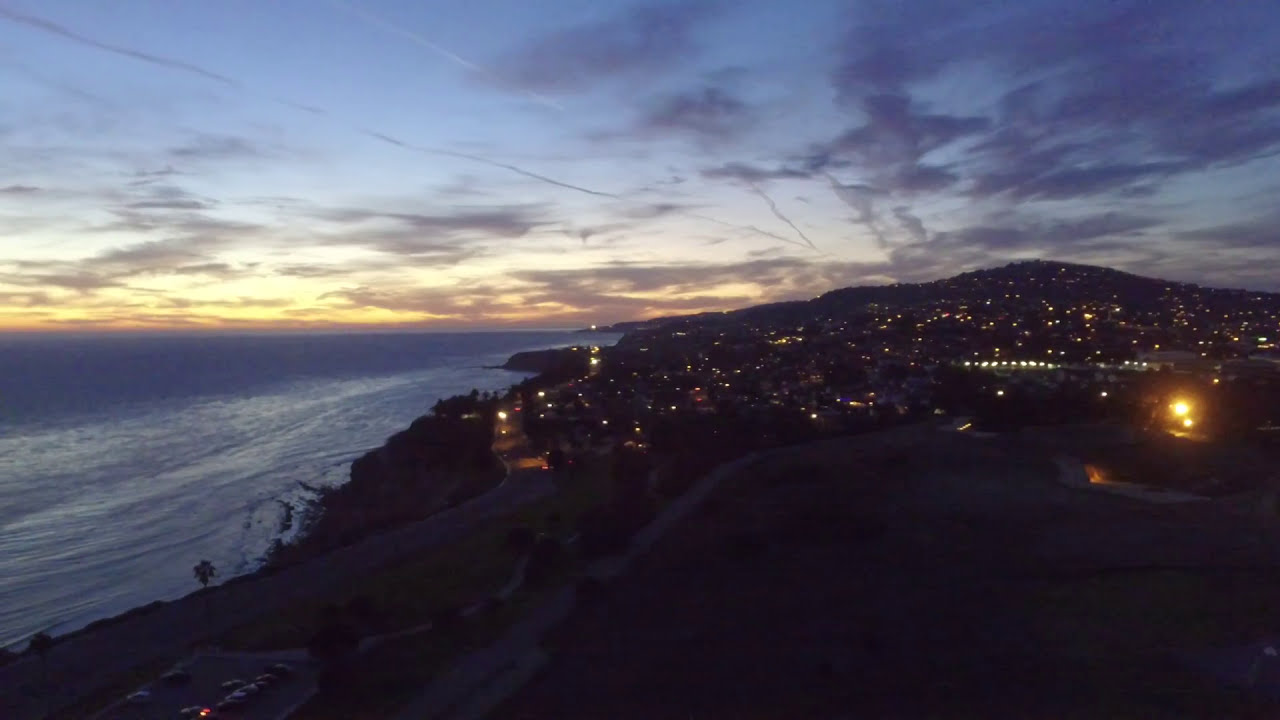In this captivating photograph taken at late sunset, the scene captures the transition to nightfall. The sun, mostly set, leaves a hint of orange on the horizon, casting a golden-yellow and orange glow across the sky. Wispy cirrus clouds hang above, gradually shifting from white to gray, and finally to dark indigo as they stretch higher into the darkening blue sky. Below the sky's gradient of colors, a serene body of water spreads out on the left, its waves gently rolling onto the shore. The water closer to the shore retains a lighter blue hue, even as nighttime approaches, while the sea further out darkens into deeper blues.

To the right, a hillside dotted with houses becomes visible as twinkling lights start to illuminate the landscape. The detailed silhouette of the town fades into the gathering dusk, making the lights of the homes and buildings the primary features against the otherwise darkened land. The overall effect is a tranquil yet lively scene where the lights of human habitation merge seamlessly with the natural beauty of the descending night.